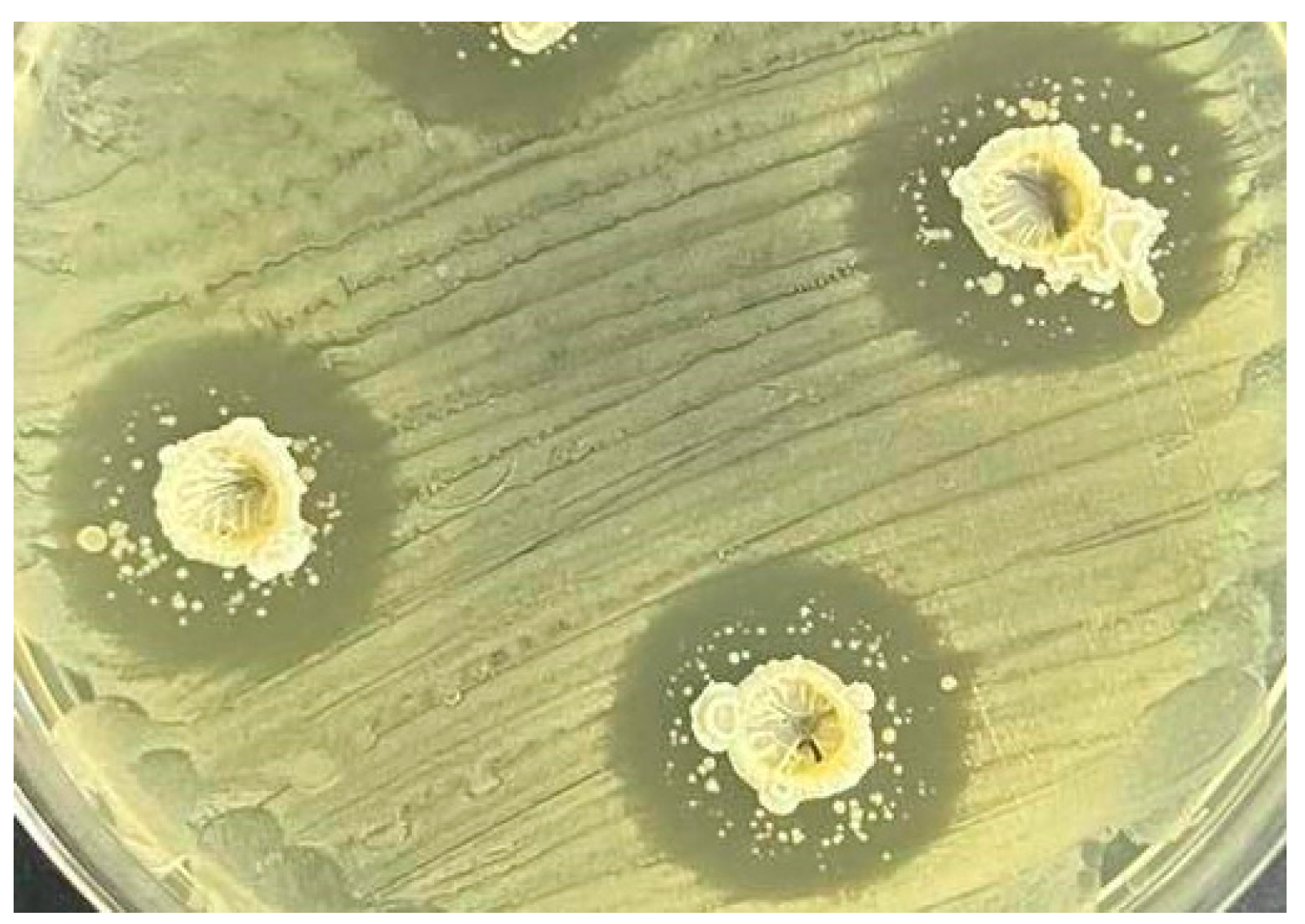The image depicts a zoomed-in view, possibly taken through a microscope, of a clear, round, glass Petri dish commonly used in laboratory settings. The dish features a blend of green and yellow colors, with irregular, dark lines resembling the grain of a wooden table, giving it an aged or weathered appearance. Within the dish, there are four distinct sections where growth-like formations are evident. These sections each contain splotches that range from light green to darker green, with a central area in each that is white or yellow, reminiscent of either small blooms or bubbles, appearing almost like microscopic flowers or bacterial colonies. The dish’s border is visibly circular and clear, creating a stark contrast with the darker, external background, and across the dish are streaks or paint-like strokes in the same green and yellow hues, adding to the intricate and somewhat organic pattern of the image.